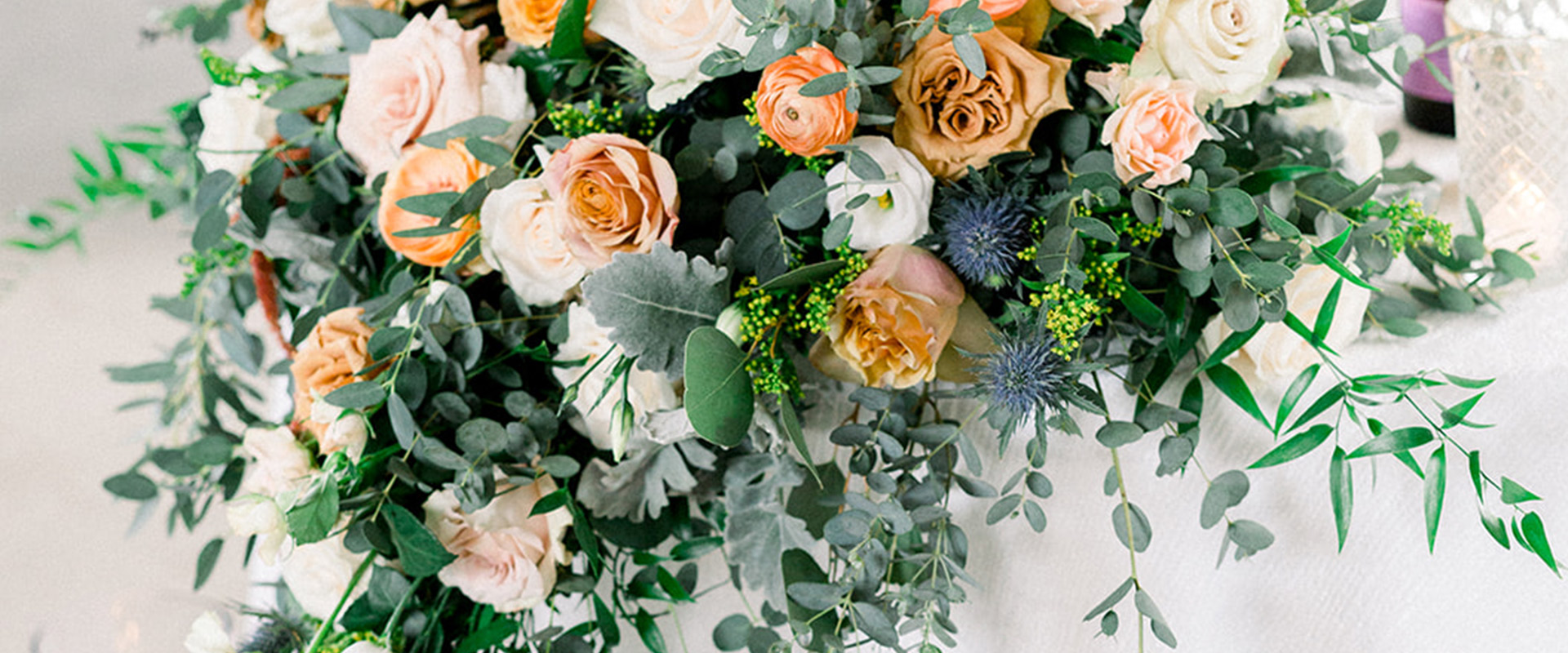The photograph showcases an elegant floral arrangement set on a flat white surface draped with a thin white fabric. The bouquet features a harmonious mix of roses in various colors, including pink, orange, gray, and white. Interspersed among the roses are smaller blue flowers and diminutive yellow buds that create a dotted effect along their stems. The entire arrangement is complemented by leafy green stems, adding a decorative and natural touch to the composition. In the top right corner of the image, a drinking glass adorned with a white latticework design can be seen, alongside a purple cylinder with a black base, hinting at additional decorative elements on the table. The overall theme of the arrangement blends shades of white, cream, peach, and orange with touches of green foliage, contributing to a sophisticated and natural-looking bouquet.